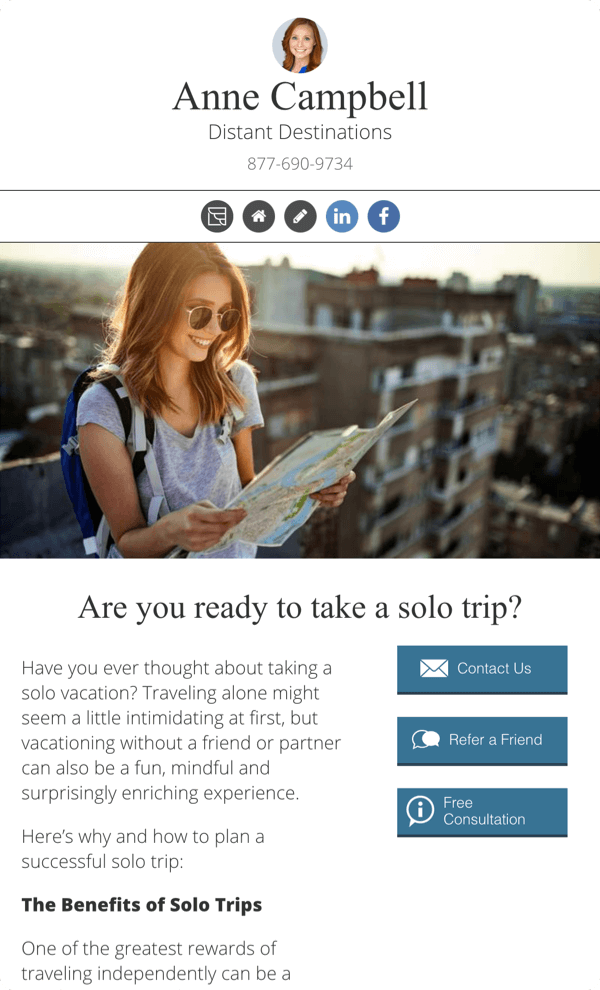In the image, a woman named Ann Campbell appears at the top. She has striking red hair and is smiling warmly, wearing glasses and a backpack. The scenery behind her includes a housing complex and a clear sky. Next to the image, text promotes solo travel with the headline "Are you ready to take a solo trip?" followed by various action prompts: "Contact us," "Refer a friend," and "Free consultation." The text continues, encouraging the idea of solo vacations, stating that although traveling alone might seem intimidating at first, it can also be fun, mindful, and surprising. Additional text outlines benefits and planning tips for solo trips, acknowledging that traveling independently offers significant rewards. Below, contact information is provided: "Distant Destinations, 877-690-9734." Icons for LinkedIn and Facebook appear, along with illustrations of circles and a pen, further adding to the inviting and informative layout.